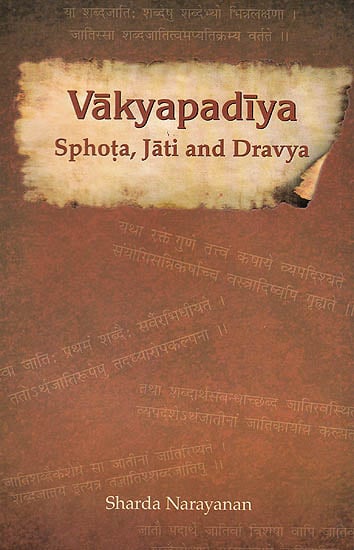The image is a detailed close-up of a book jacket, primarily in brown with an intentionally worn-looking design. The background features a dark orange to brown gradient with faint lines of text in what appears to be Arabic, creating an antique effect. Prominently in the upper half, there is a piece of parchment paper with burnt and weathered edges, giving the title clearly in bold brown print: "Vakya Padiya." Below the title, additional terms are listed: "Svota," "Jati," and "Dravya." Scattered throughout the cover are very faint lines of text in a lighter brown shade, suggesting fragments of another language. The author's name, "Sharda Niranjanan," is written in yellow at the bottom of the cover. The image is well-lit and clearly showcases the intricate design elements of the book jacket.